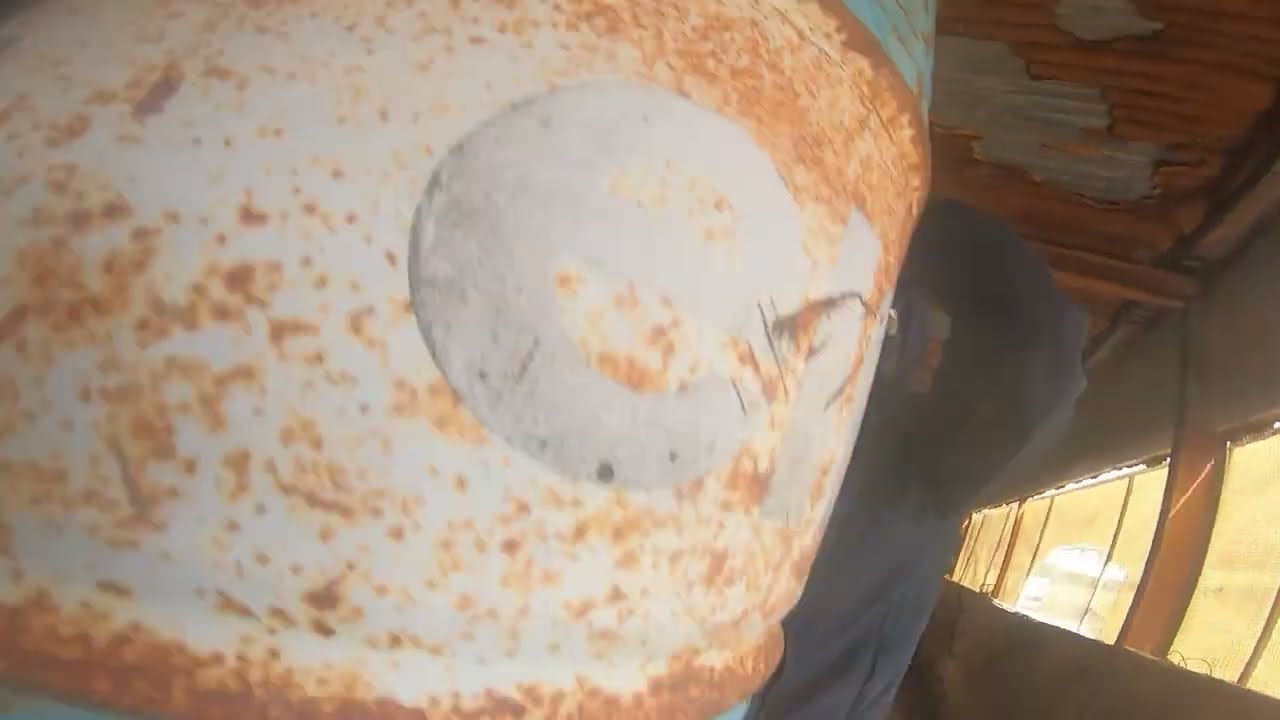This image is a close-up, color photograph taken indoors, depicting a large, cylindrical metal object prominently occupying the left two-thirds of the frame. Initially painted white, the object is heavily rusted with brown and orange streaks and spots, suggesting extensive exposure to moisture, possibly seawater. A white, circular knob protrudes slightly from the object's center, adding a tactile element to its weathered surface. The top section of the object sports a faded teal hue, further contributing to its worn appearance.

To the right of this rusted canister or drum, we see part of a wall featuring a series of long windows, covered with beige or light-yellow shades that emit a soft, ambient light. Against this background, a person wearing a gray jacket is partially visible; they appear to be standing or moving to the right, with only their upper torso and left arm discernible. Above, the ceiling is made of corrugated metal, displaying two distinct layers: a deteriorating, rusted brown layer below and a more intact gray layer above. The ceiling shows signs of peeling and decay, mirroring the overall rustic and neglected aesthetic of the scene.